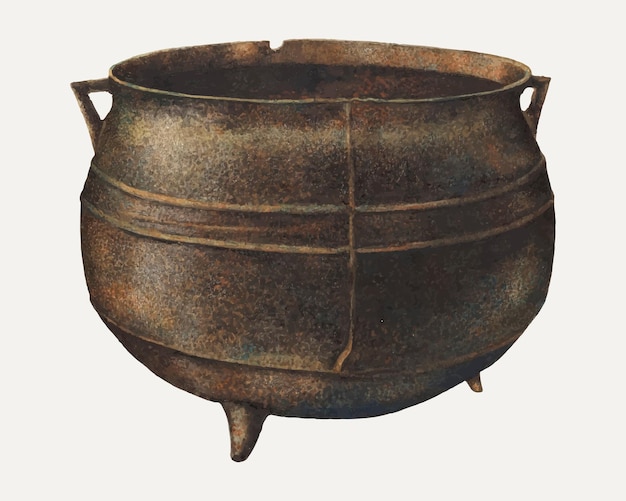This image showcases a detailed drawing or painting of an old cast-iron cauldron, depicted in varying shades of brass, black, and rusty brown. The cauldron, prominently centered against a light gray to off-white background, appears to be floating. It features a round shape with an open top and has distinct welding details, including a vertical seam running down the side, and two parallel horizontal lines that encircle it. Notably, there are triangular-shaped handles on both the left and right sides. The cauldron stands on three triangular legs, although only two are visible in the image. Adding to its antique appearance, the piece also boasts a small cutout on the back side, designed for pouring. The combination of its patina and carefully detailed shading gives the cauldron a textured, worn look, enhancing its vintage charm.